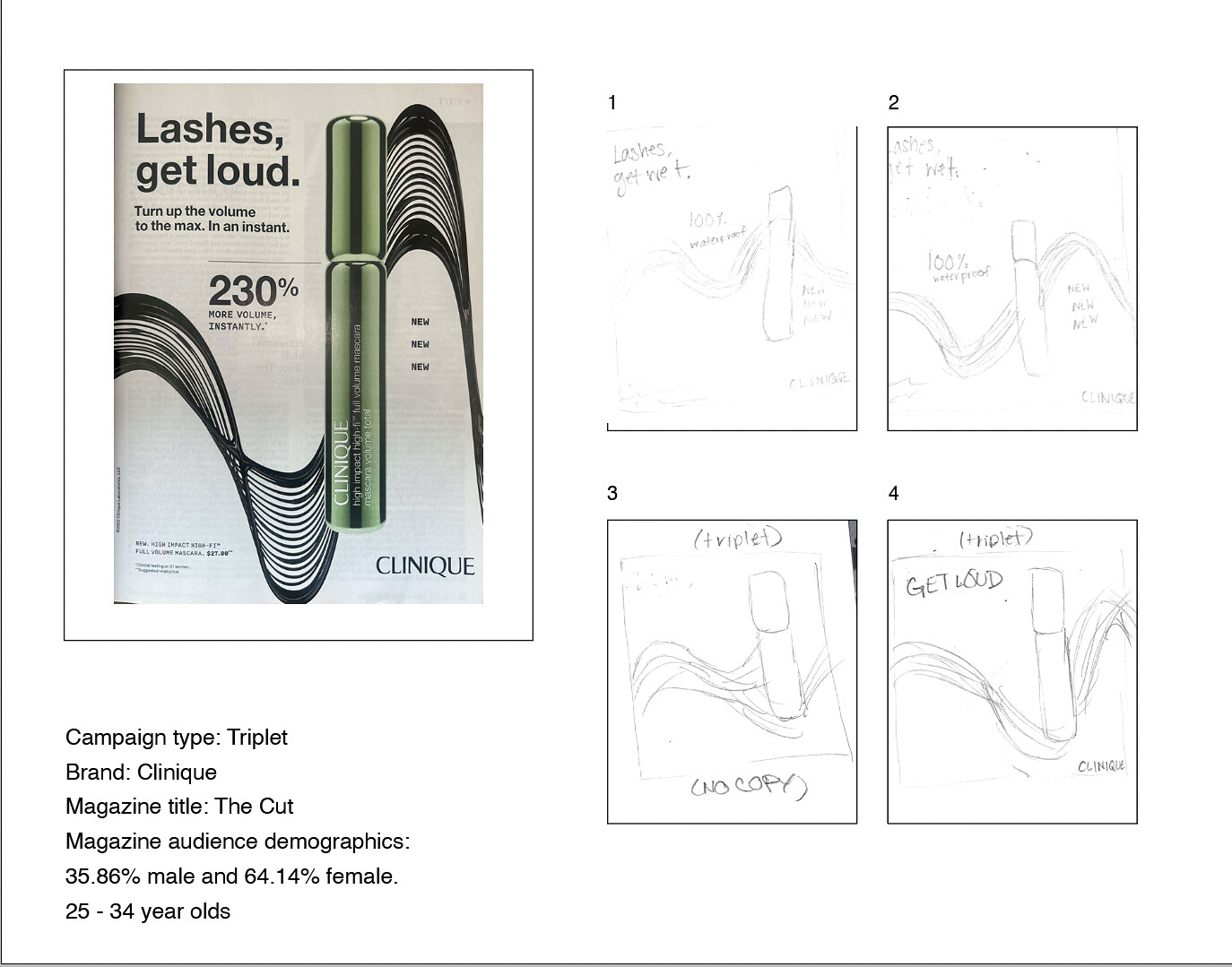The image features a graphic-styled magazine ad for a product by Clinique, specifically a full-volume mascara. Dominating the left side of the ad is a photograph of a green tube of mascara set against a black-and-white wave background, with bold text proclaiming "Lashes Out Loud, Turn Up the Volume to the Max for an Instant, 230% More Volume Instantly." The tube features the Clinique branding, and the words "new, new, new" are written beside it. 

To the right of the main image, there are four sequential panels numbered 1 to 4, each containing hand-drawn sketches of the original ad. Panel 1 features the phrase "lashes get wet, 100% manageable," while panel 2 reiterates "lashes get wet, 100% waterproof, new, new, new, Clinique." Panels 3 and 4 contain text such as "triplet, no copy," and "triplet, get loud, Clinique," suggesting these sketches illustrate the creation process of the ad. 

In the bottom left corner of the ad, additional text provides campaign details: "Campaign Type: Triplet, Brand: Clinique, Magazine Title: The Cut, Magazine Audience: 35.86% male and 64.14% female, aged 25-34."